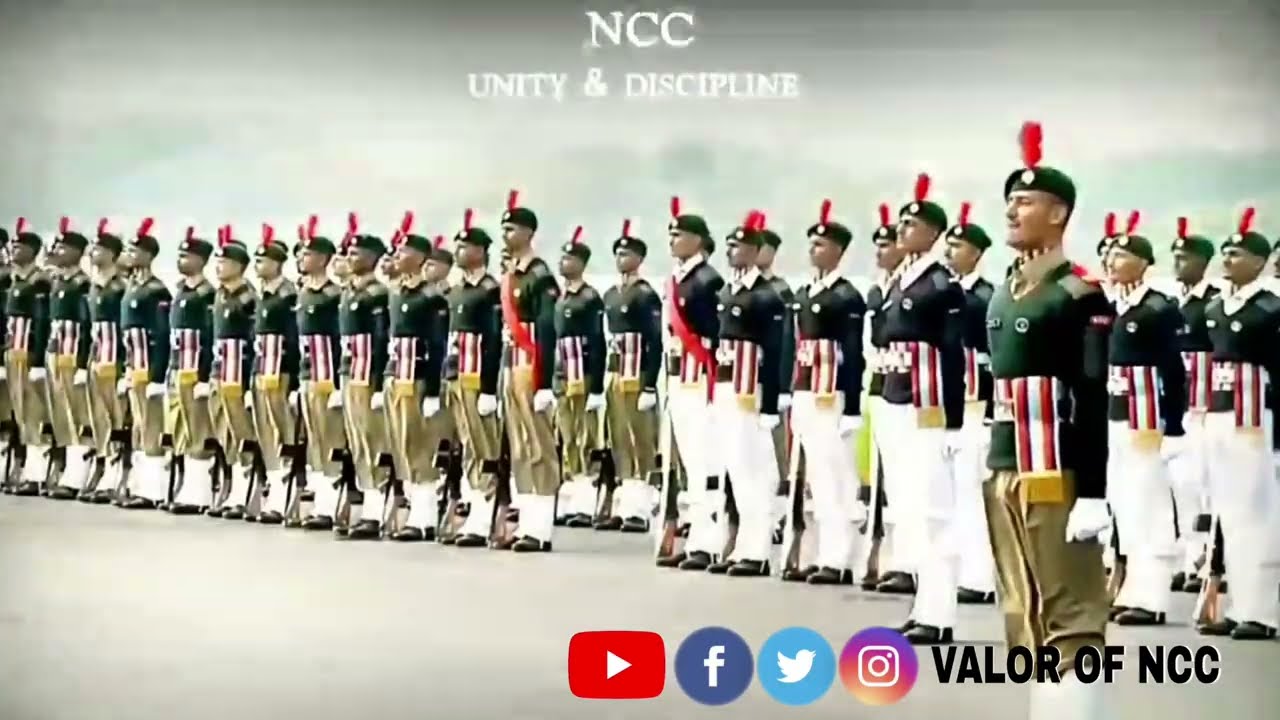The image depicts a platoon of uniformed soldiers standing in formation. These soldiers, likely from another country, are dressed in dark green sweaters and green berets adorned with red feathers and white badges. Some wear white pants while others are clad in khaki or tan pants, and all have black boots with white protectors over their trousers. Many soldiers feature diagonal ribbons across their chests and all hold rifles with stocks grounded, barrels pointed upward.

An officer, presumably the commander, stands at the front of the group, distinguished by his white gloves. The backdrop has a light gray overcast ambiance, accentuating the soldiers’ attire. At the top center of the image, the text "NCC, Unity and Discipline" is displayed in white lettering, while the bottom right corner features the phrase "Valor of NCC." Additionally, the logos for social media platforms YouTube, Facebook, Twitter, and Instagram are visible to the left of the bottom text, indicating that this might be a screenshot or a designed poster. The sky in the background has a blue-green hue, enhancing the overall composition of the military scene.